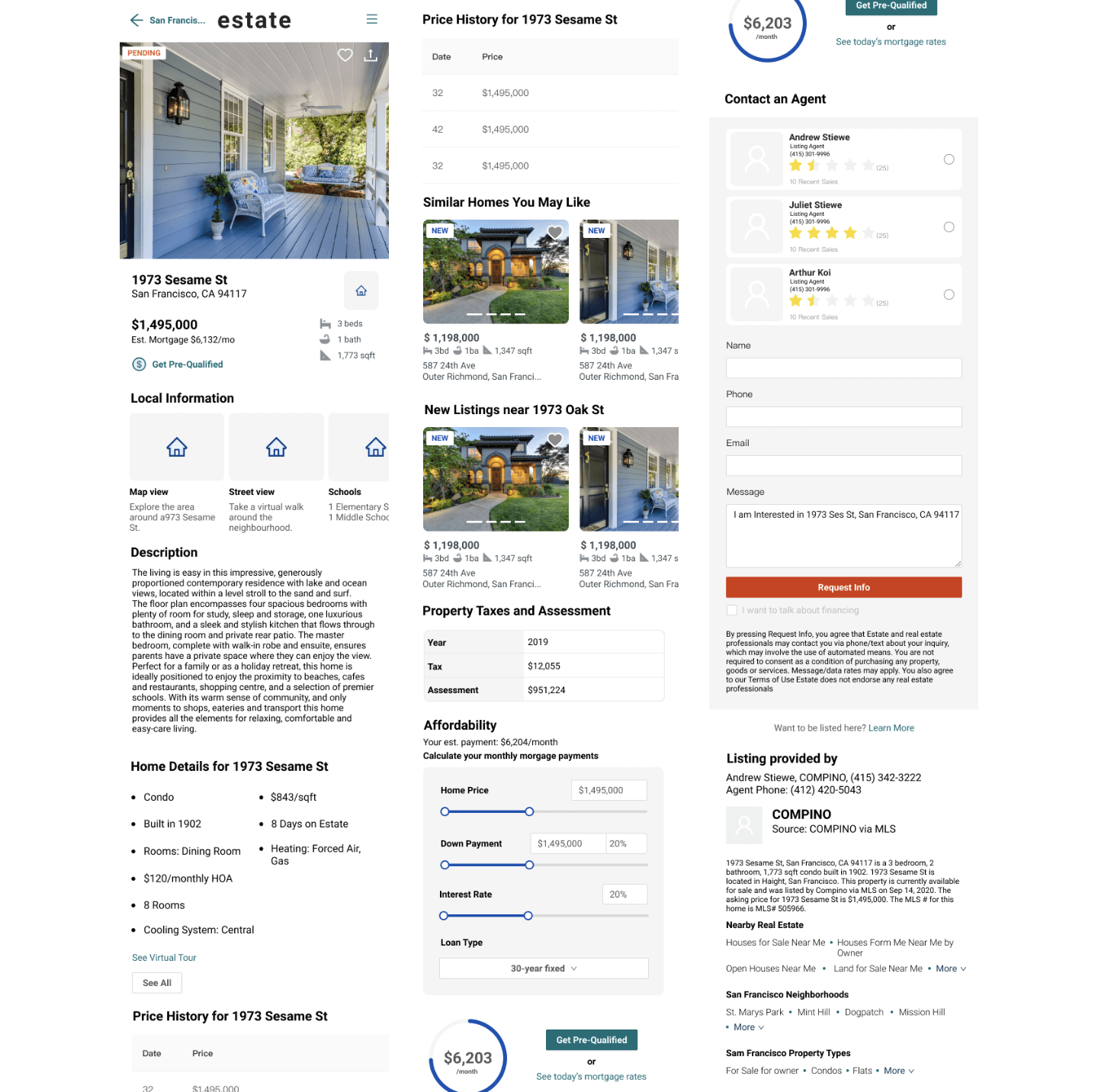This screenshot features a detailed listing from what appears to be a real estate website. The primary image in the upper left corner showcases a charming front porch, painted in vivid blue hues. The porch walls and floorboards are uniformly colored, creating a cohesive and inviting aesthetic. Adorning the porch is an assortment of furniture, including a loveseat positioned towards the back, with lush foliage visible just behind it, adding a touch of greenery and tranquility. Near a blue-painted window, a chair is thoughtfully placed next to a potted plant, enhancing the cozy, homely atmosphere.

Adjacent to the porch image is a segment labeled 'Price History,' displaying a list of previous prices for the property, though the specific numbers are too small to discern clearly. The address, presumably located at 1973 Sesame Street, is also mentioned in diminutive text.

Beneath the price history section, there is a collection of recommended similar homes. Highlighted among them is an image of a house flanked by verdant foliage on both sides. The photo captures the front view of the house, featuring a pathway or driveway leading directly to the front door, inviting potential buyers to envision their future in this picturesque setting.